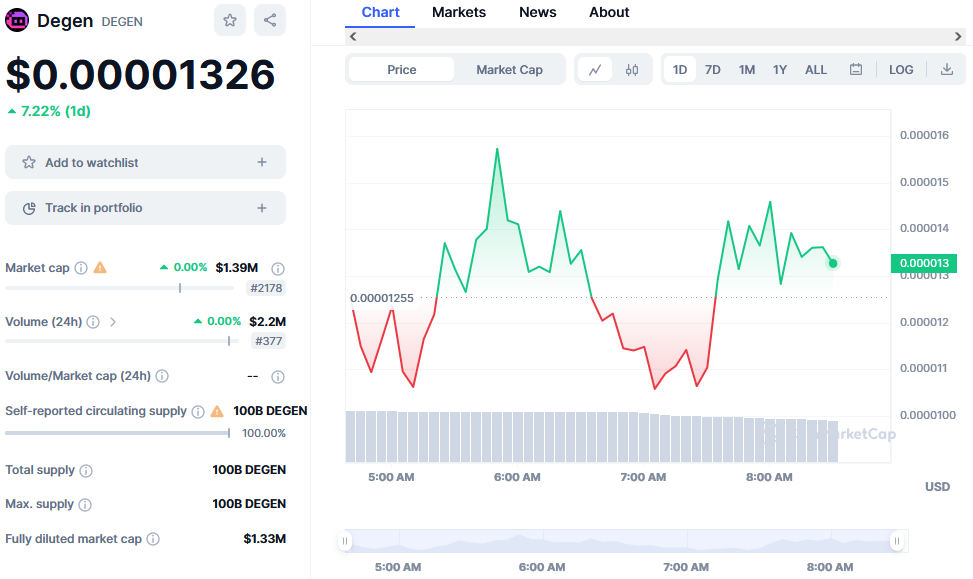A cryptocurrency called Degen (D-E-G-E-N) currently has a value of $0.00001326 per coin, reflecting a 7.22% increase over the past 24 hours. The image shows detailed information on the left pane, including metrics such as market cap ($1.39 million) and trading volume. On the right, a graph illustrates the coin's fluctuating trend throughout the day, with notable peaks and troughs; initially dipping before experiencing a series of rises and falls. The watermark at the bottom right suggests the data is sourced from CoinMarketCap. Additionally, options to adjust the time range and search for related news and market information are also visible. As typical for new cryptocurrencies with a vast number of coins in circulation and minimal individual value, even minor increases can result in significant percentage gains.